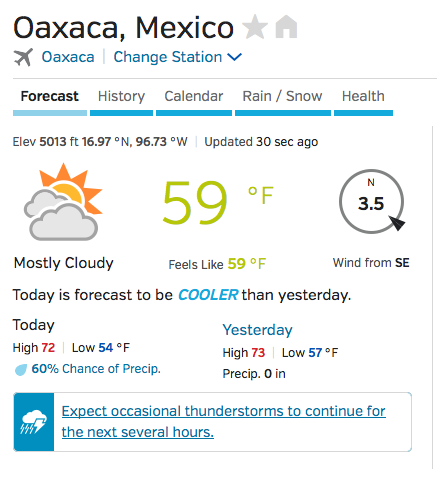This detailed caption corresponds to an image of a weather forecast for Oaxaca, Mexico. The forecast is presented on a white background with most text in blue or black.

**Top Section:**
- In bold black letters at the top: "Oaxaca, Mexico."
- Adjacent to the location name: a gray star shape, followed by a gray house shape.
- Below it, a series of symbols and text with mixed colors: a gray airplane icon next to "Oaxaca" in blue, a vertical gray line, "Change Station" in blue, and a blue downward-facing caret symbol.
- A thin horizontal gray line below this section separates the header from the forecast details.

**Navigation Tabs:**
- Below the gray line, a series of tabs for navigating different forecast features: "Forecast" in black with a light blue rectangle underneath it, followed by "History," "Calendar," "Rain/Snow," and "Health," all in black text with darker blue rectangles beneath each.

**Forecast Details:**
- The forecast details include geographical and meteorological information in black text:
  - "Elevation 5,013 feet, 16.97° N, 96.73° W, updated 30 seconds ago."
- The current weather condition is shown:
  - Temperature: "59°F" in green.
  - A sun icon with gray clouds indicating "Mostly Cloudy" in black text below it.
  - Wind information on the right: a gray circle with “North 3.5” and "Wind from Southeast" inside.

**Additional Weather Details:**
- Wind chill value: "Feels like 59°F."
- Comparison of today's and yesterday’s weather:
  - "Today is forecast to be cooler than yesterday."
  - "Today: High 72, Low 54."
  - "Yesterday: High 73, Low 57."
- A forecast note: "Expect occasional thunderstorms to continue for the next several hours."